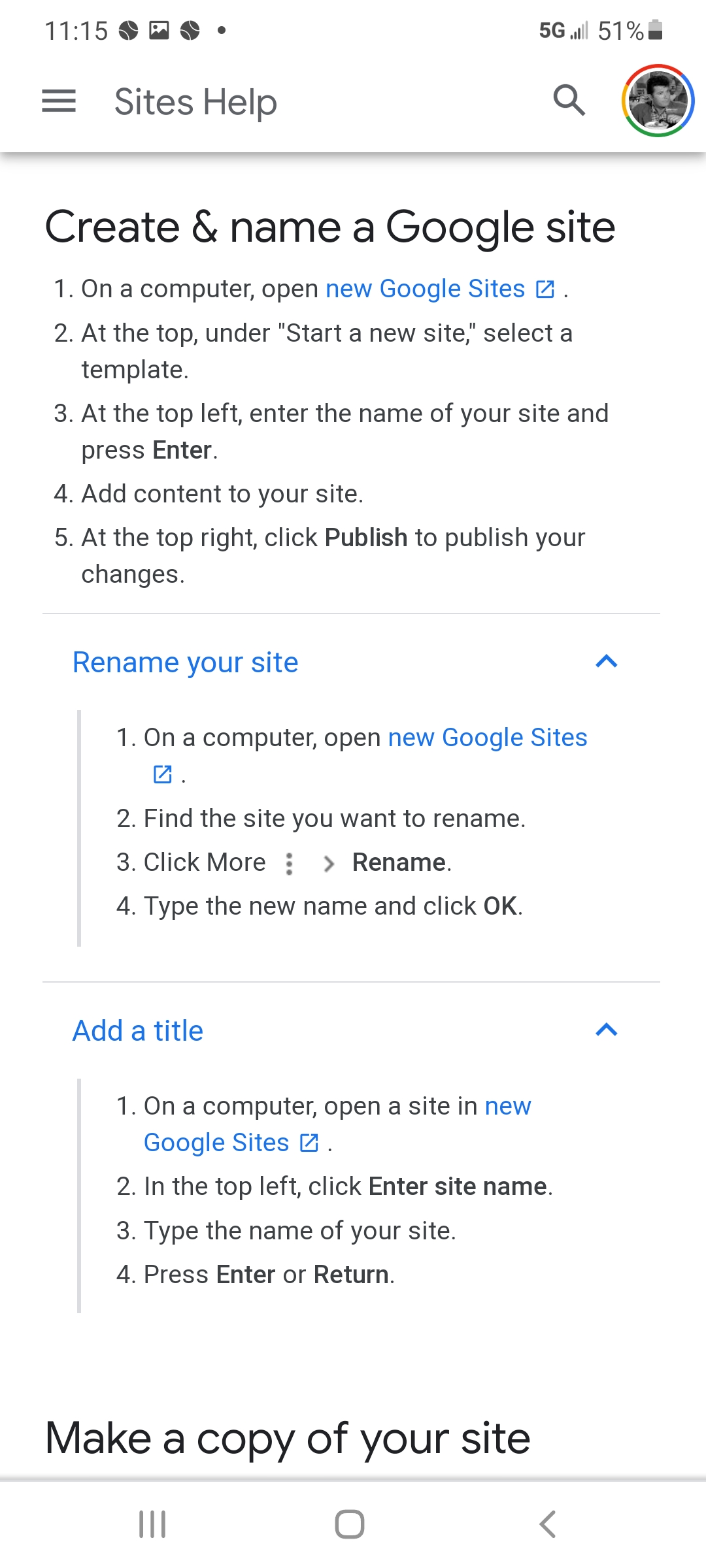The image is a vertical rectangle, resembling a screenshot from a Google application on a smartphone. At the top left of the image, there is a black text displaying the time "11:15" along with several standard smartphone icons. Below that, in gray text, it says "Sites Help," followed by "Create and Name a Google Site" in black text.

The image details five steps to create and name a Google Site:
1. On a computer, open New Google Sites.
2. At the top, under "Start a new site," select a template.
3. At the top left, enter the name of your site and press Enter.
4. Add content to your site.
5. At the top right, click "Publish" to publish your changes.

All hyperlinks in this section are blue. Below these instructions, the image provides a guide titled "Rename Your Site," also in blue text, with the following steps:
1. On a computer, open New Google Sites.
2. Find the site you want to rename.
3. Click "More" (indicated by an arrow), then "Rename."
4. Type the new name and click OK.

Similar blue hyperlinks are used for "Rename your site" and "New Google Sites." Further down, there's another section in blue text titled "Add a Title," with four steps:
1. On a computer, open a site in New Google Sites.
2. In the top left, click "Enter site name."
3. Type the name of your site.
4. Press Enter or Return.

At the very bottom, in black text, it states "Make a Copy of Your Site," with corresponding blue links for "Add a Title" and "New Google Sites." The entire background of the image is white, reinforcing its appearance as a straightforward screenshot from a smartphone application.